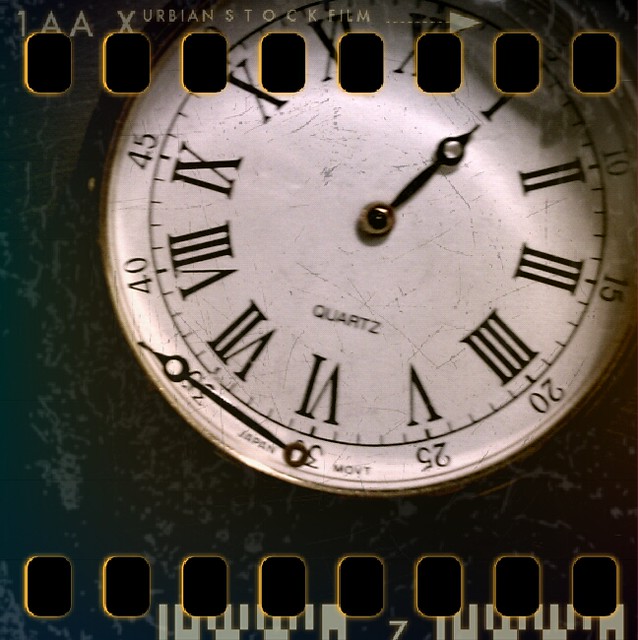The photograph captures a vintage clock with a white face adorned with Roman numerals from I to XII. The clock is positioned at an angle, with the numeral XI nearly at the top, slightly to the left of center. The face is marked by noticeable cracks, adding to its aged appearance. The word "QUARTZ" is inscribed beneath the XII, and at the bottom of the clock face, the words "JAPAN MOV'T" are visible. The hour hand is intact and points to I, while the minute hand has detached and rests at the bottom, both hands colored black. The clock is set against a gray background, marred by smudges and light gray spots. At the top of the image, "1AAXURBIAN STOCK FILM" is printed, flanked by eight perforations resembling those found in old film strips, mirrored by an identical set at the bottom.